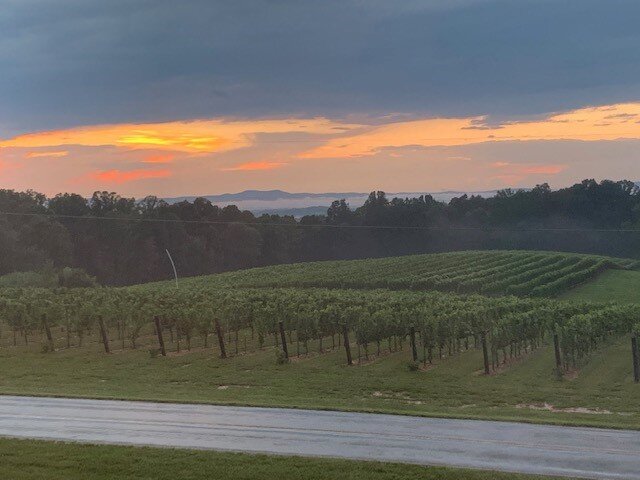The image depicts a sunset scene viewed through the window of a vehicle, potentially a train, bus, or car, adding a grey hazy cast to the picture. The foreground showcases a paved road running horizontally across the frame, bordered by a strip of grass. Beyond the road lies a sprawling vineyard with rows upon rows of grapevines that stretch all the way to a distant tree line. The vineyard appears lush and green, despite the absence of visible fruit on the vines. As the eye moves further back, the sky transitions from a dark hue at the top to a warm orange near the horizon, highlighting the sun's descent. The silhouettes of dark trees and faint outlines of distant mountains shrouded in fog create a serene and somewhat mystical background, enhancing the overall tranquility of the sunset-lit landscape.